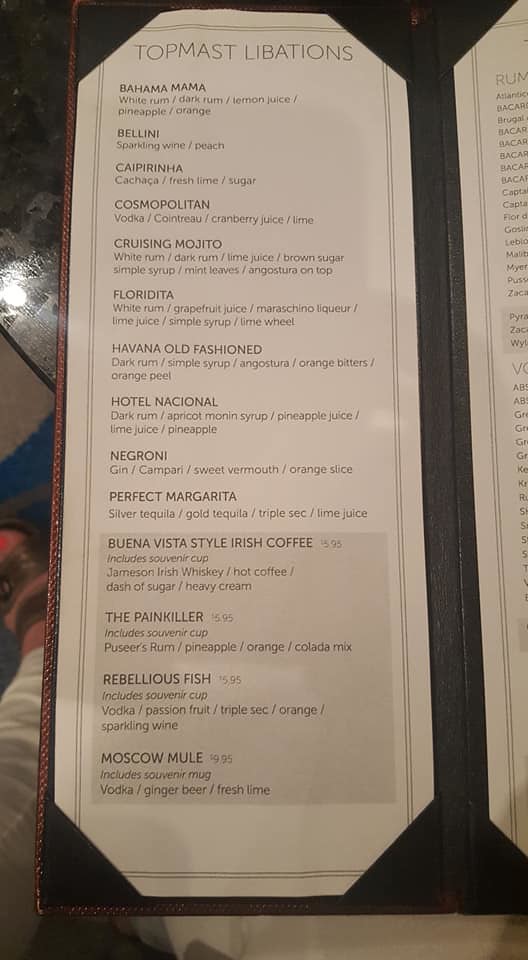A close-up image displays a sleek, black leather menu holder featuring a meticulously tucked, pristine white page with elegantly dark-colored font. The top and bottom corners of the menu holder are subtly visible, securing the paper in place. The header reads "Top Mask Libations," introducing a curated list of enticing beverages. Each drink is detailed with its ingredients as follows:

- **Bahama Mama**: White Rum, Dark Rum, Lemon Juice, Pineapple, Orange
- **Bellini**: Sparkling Wine, Peach
- **Caipirinha**: Cachaça, Fresh Lime, Sugar
- **Cosmopolitan**: Vodka, Cointreau, Cranberry Juice, Lime
- **Classic Mojito**: White Rum, Dark Rum, Lime Juice, Brown Sugar, Simple Syrup, Mint Leaf, Angostura Bitters
- **Floridita**: White Rum, Grapefruit Juice, Maraschino Liqueur, Lime Juice, Lime Syrup, Lime Wheel
- **Havana Old Fashioned**: Dark Rum, Simple Syrup, Angostura Bitters, Orange Bitters, Orange Peel

Additional drink names, such as Hotel Nacional, Negroni, Perfect Margarita, Buena Vista-style Irish Coffee, The Painkiller, Rebellious Fish, and the Moscow Mule, are listed further down, with their respective ingredients detailed underneath each entry. The overall presentation is refined, catering to an elegant dining or bar atmosphere.